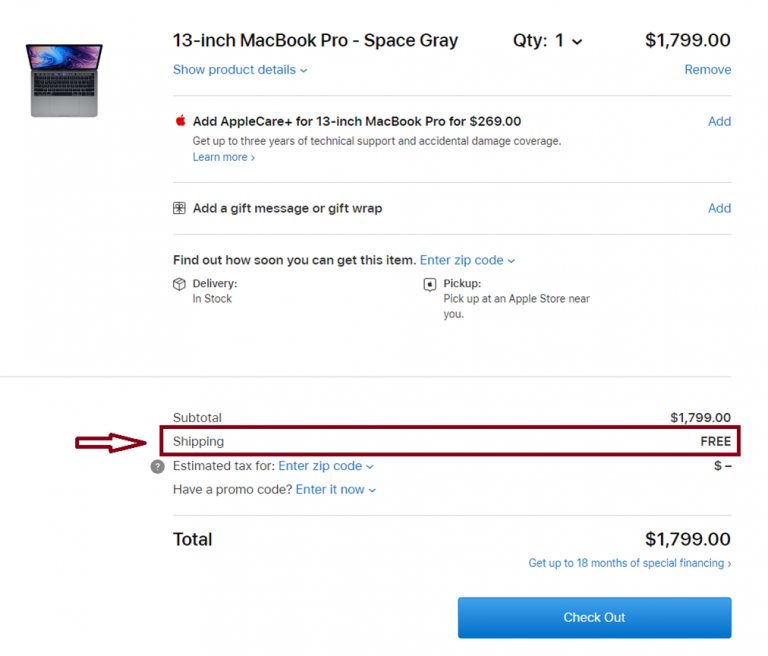The webpage features an online listing for a MacBook Pro in an organized horizontal layout with no outer border and a white background.

**Image Section:**
- **Position:** Upper left corner.
- **Details:** The image shows an open MacBook Pro from a slightly top-down angle. The display, only partially visible, features a colorful abstract pattern. The focus is on the silver chassis and black keyboard of the laptop.

**Text and Sections:**

1. **Top Section:**
   - **Title:** "13-inch MacBook Pro – Space Gray" in bold, dark gray, left-justified text.
   - **Quantity:** "QTY: 1" with a dropdown arrow for adjustment.
   - **Price:** "$1,799.00," right-justified.
   - **Options:** Beneath the price, "Remove" in blue, right-justified text. Below the title, "Show product details" with a downward-facing arrow to click for details.
   - **Divider:** A horizontal light-gray underline.

2. **AppleCare+ Section:**
   - **Logo:** A red Apple logo in the upper left.
   - **Text:**
     - In bold, "Add AppleCare+ for 13-inch MacBook Pro for $269.00".
     - Smaller text: "Get up to three years of technical support and accidental damage coverage."
     - "Learn more" in blue with a right-facing arrow for additional information.
   - **Link:** "Add" in blue, right-justified.
   - **Divider:** Another horizontal line.

3. **Gift Wrap Section:**
   - **Icon:** A present or plus-sign logo on the left.
   - **Text:** "Add a gift message or gift wrap."
   - **Link:** "Add" in blue, right-justified.
   - **Divider:** Horizontal line.

4. **Delivery Information:**
   - **Text:**
     - "Find out how soon you can get this item" in bold black text.
     - "Enter zip code" in blue with a dropdown arrow for availability.
   - **Details:**
     - Delivery: "Delivery: In Stock" with a box icon.
     - Pickup: "Pick up at an Apple Store near you" with an Apple Store icon.
   - **Divider:** A horizontal gray line.

**Pricing Summary:**
- **Sub-total:** "Subtotal: $1,799.00," listed first.
- **Shipping:** "Shipping: FREE," highlighted with a red box, and red outlined arrow pointing towards it.
- **Estimated Tax:** "Estimated tax for:" with a gray question mark icon, "Enter zip code" in blue with a dropdown arrow. The tax amount is not calculated without the zip code.

**Promo Code Section:**
- **Text:** "Have a promo code?" prompt.

**Final Total:**
- **Text:**
   - "Total: $1,799.00" in left-justified text.
   - "Get up to 18 months of special financing" followed by a blue right-facing arrow.
- **Checkout Button:**
   - A blue rectangular button with rounded corners, centrally labeled "Checkout" in white text.